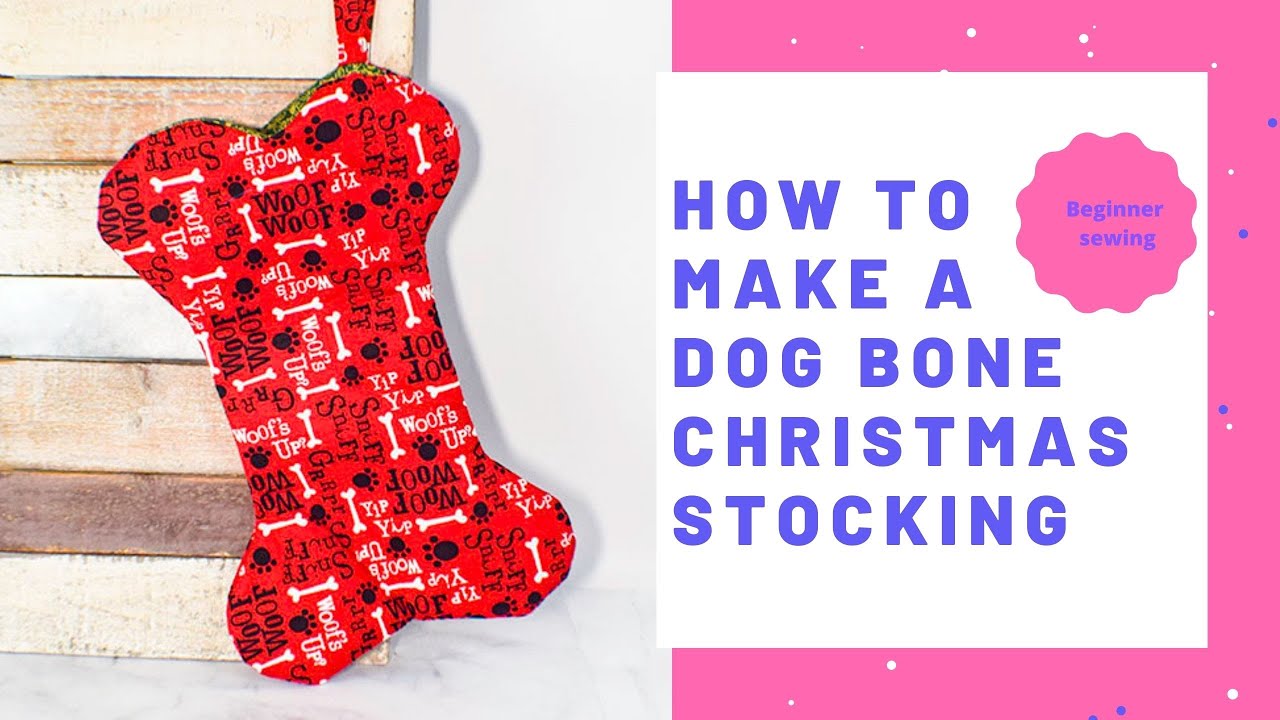This social media graphic is a detailed tutorial on making a dog bone-shaped Christmas stocking. The image is split; on the left side, there is a red bone-shaped stocking adorned with a black and white detail. The stocking features playful phrases such as "woof woof," "woofs up," "sniff sniff," along with paw prints and bone illustrations. The stocking is paired with a matching red fabric hanger patterned similarly. The background includes various colored wood planks and a white wall, adding to the festive atmosphere.

The right side of the image has a pink background with a white overlay, where purple text reads "How to Make a Dog Bone Christmas Stocking." The text is framed by a pink border decorated with white and blue dots. In the top right corner, an octagon with a squiggly pink outline and blue text signifies that this is a "Beginner Sewing" project, making it clear that this is an accessible and fun DIY activity.